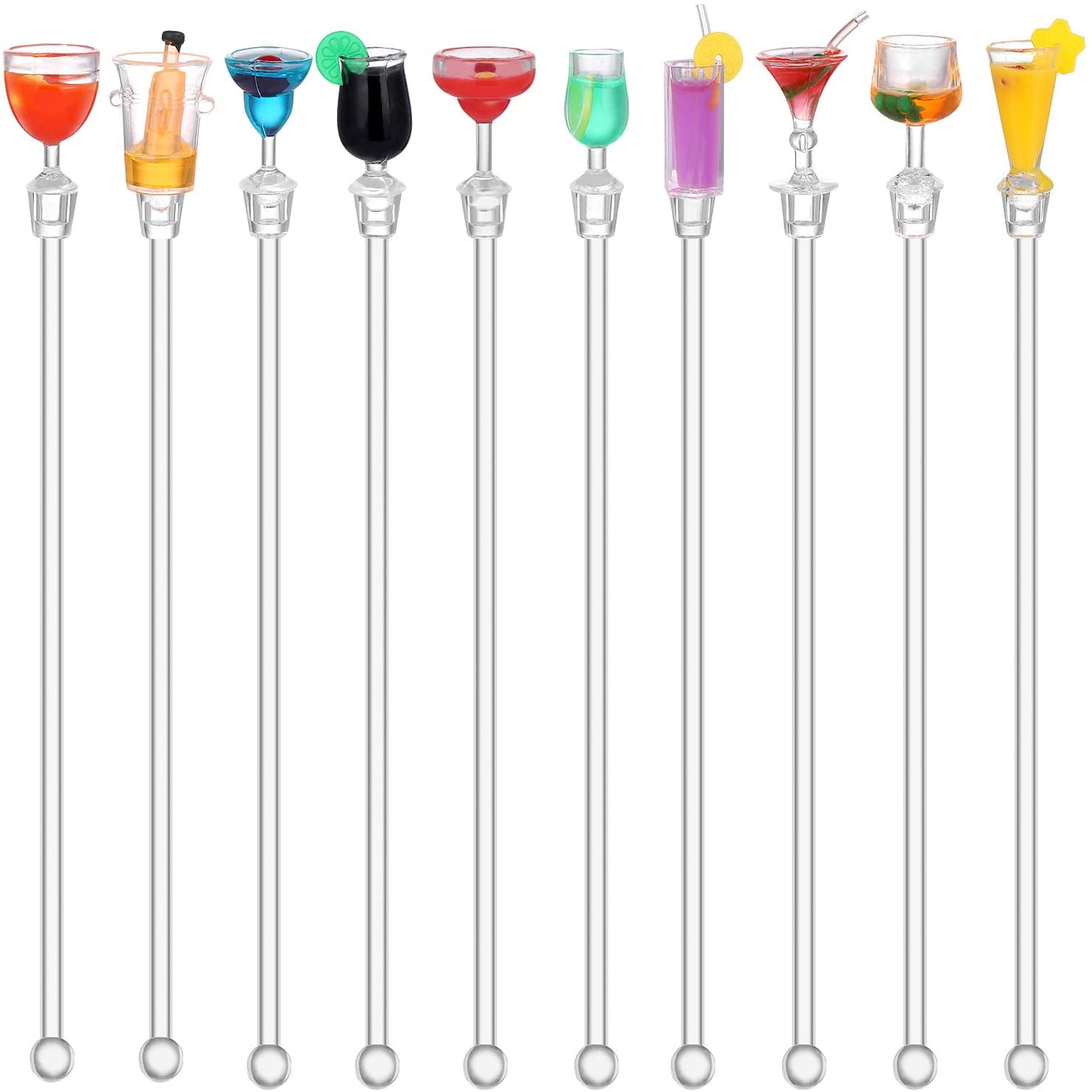This image features a collection of ten distinct mixed drinks, each presented in a unique glass perched atop long, gray vertical rods. The rods have small, light gray circles at their bases, outlined in a darker gray. Each drink container has a specific design and color, capturing the essence of a diverse array of cocktails against a plain white background without any text or borders.

Starting from the left, the first drink is in a short-stemmed glass filled with orange liquid. Moving right, the next container appears to hold gold liquid with a black-topped object submerged within it. The third drink is in a glass with a slightly longer stem, containing blue liquid. The fourth glass, characterized by a very short stem, holds black liquid garnished with a lime on the rim. The fifth drink is housed in a taller-stemmed glass with a red liquid resembling a margarita. The sixth glass has bright green liquid with a small yellow object floating within it.

Continuing right, the seventh drink is in a drinking glass filled with purple liquid with a lemon on the rim. The eighth glass, in a martini shape, contains a vibrant red liquid. The ninth drink is in a wider glass that is partially filled with orange liquid and has something green floating in it. The last, and tenth, drink on the far right appears to resemble a piña colada, served in a narrow glass that widens towards the top and is filled with yellow liquid.

This playful and vibrant depiction showcases the variety and allure of mixed drinks, presented in an imaginative manner, though the rods supporting them add an element of whimsy and perplexity to the scene.